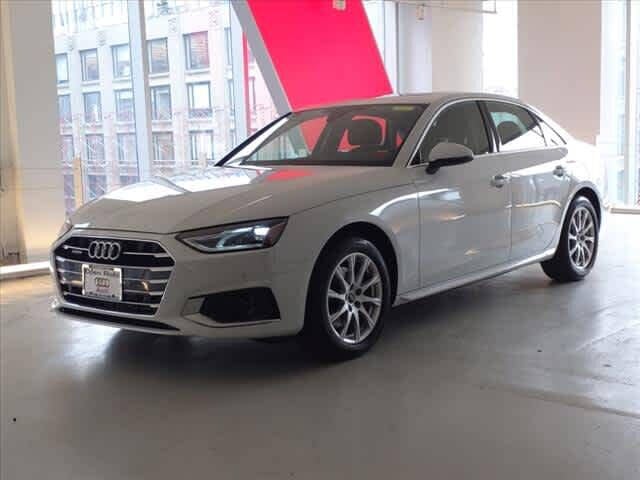The image depicts a white Audi sedan parked indoors, likely in a dealership showroom rather than a parking garage, as it has no license plate. The car is viewed from a front diagonal angle, showing both the front and driver’s side. The distinctive Audi emblem with four rings is prominently displayed on the front grille, while the headlights are flat and sleek. The Audi features four doors and is positioned over a light gray cement floor.

Surrounding the vehicle, the setting includes off-white walls and a backdrop featuring windows that reveal a neighboring high-rise building. There is a noticeable pink strip that trims this high-rise window. Additionally, the light filtering in through these windows casts reflections on the car's shiny surface, creating a subtle shadow that gives it a light gray appearance despite its true white color. The tires are equipped with silver spoke rims, and the driver’s side rearview mirror is light gray on top and black on the bottom.